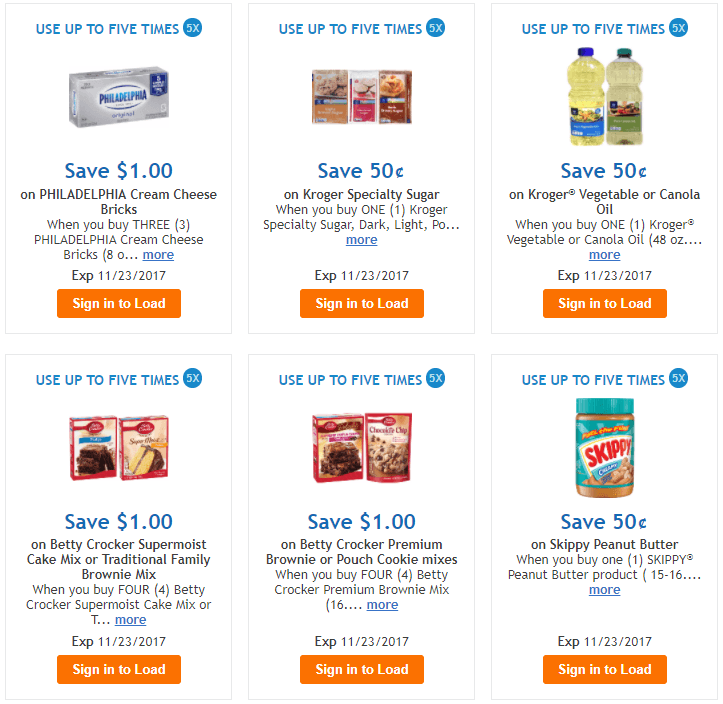This advertisement showcases a variety of grocery store sale items and coupon offers. In the upper left corner, there is a promotion for Philadelphia Cream Cheese, allowing customers to save $1.00. Adjacent to it, in the upper middle, is a deal for Kroger Specialty Sugar, offering savings of $0.50 when you buy one. The advertisement prompts shoppers to sign in to load the coupon, valid until November 23, 2017. In the upper right corner, a similar offer is presented for Kroger Vegetable or Canola Oil, with a $0.50 discount, also requiring a sign-in to load.

In the lower left section, the advertisement highlights a savings opportunity of $1.00 on Betty Crocker Super Moist Cake Mix or Traditional Family Brownie Mix, again expiring on November 23, 2017. Directly below, there is a promotional offer for Betty Crocker Premium Brownie or Pouch Cookie Mixes, where buying four entitles you to a $1.00 savings, applicable up to five times per customer. The notification to sign in to load this coupon is emphasized in an orange box.

Finally, in the lower right corner, the ad features a $0.50 savings on Skippy Peanut Butter when purchased, with a visual of the Skippy product included. This coupon can be used up to five times, stated in blue text, and also requires sign-in to access.

Each offer within this advertisement provides the added convenience of digital coupons, encouraging customers to sign in to the store's system to load the savings, which are valid until November 23, 2017.